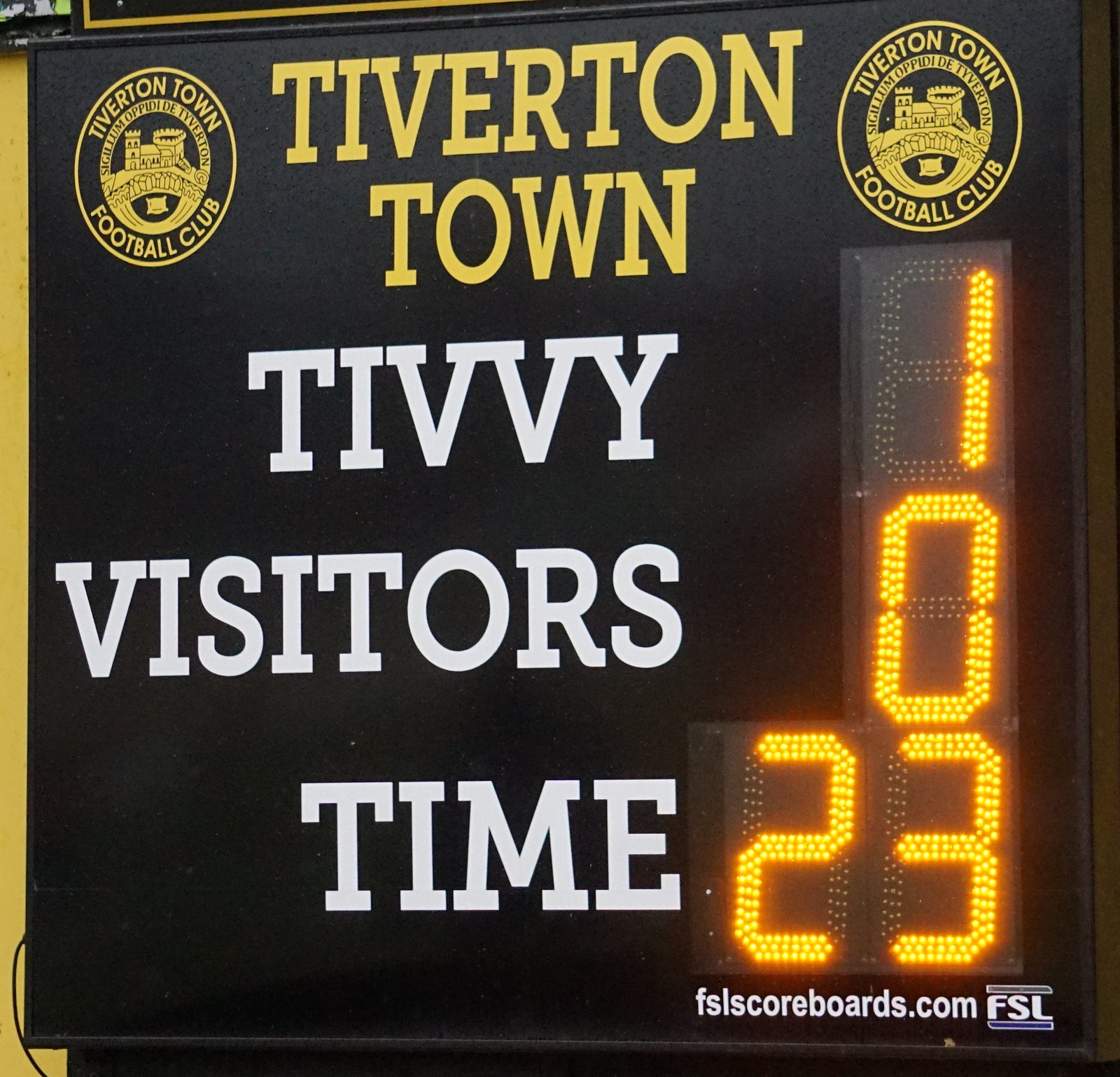The image showcases a digital scoreboard from Tiverton Town's ground, prominently featuring a black background with striking yellow accents. At the top center, the bold yellow capital letters spell out "TIVERTON TOWN." Flanking this heading are two identical logos, each featuring a yellow-golden circular seal with an outermost ring and an innermost circle. The area between the rings is inscribed with “Tiverton Town” at the top and “Football Club” at the bottom. In the innermost circle appears an image of a castle or building, along with the name "Sigliam Opity Day Tiverton."

Below the main heading, large white capital letters display "TIVY" and "VISITORS," with the adjacent digital display indicating the score: "TV 1 VISITORS 0." Directly below, the time is displayed as "23" on the right. At the bottom right corner, a small footnote reads "FSLSCOREBOARDS.COM" with the FSL logo beside it.